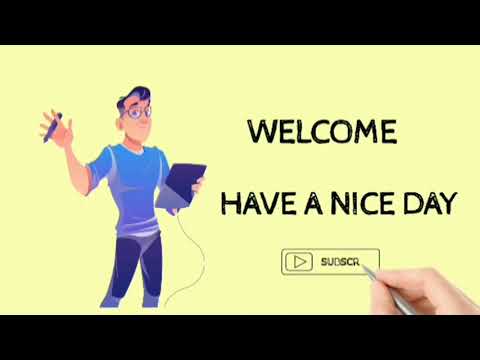The image depicts a cartoon-style illustration of a man on a slide or screenshot with a cheerful message. The scene is framed by black horizontal bars at the top and bottom, with a light yellow background in the middle. The cartoon man is positioned on the left side, wearing glasses, blue pants, and a medium blue long-sleeve shirt rolled up to his elbows. He has medium to light skin and black hair that may be slightly graying. In his right hand, he holds a pen or possibly a blue writing instrument, while his left hand holds what appears to be an iPad attached to a cable or paracord. To the right of the man, in bold black capital letters, are the words "WELCOME" followed by "HAVE A NICE DAY." Below this text, a hand is seen using an Apple pencil to manually draw the YouTube subscribe button, which is currently incomplete, showing only as far as the letter 'R' in "SUBSCRIBE" and not yet colored in red.